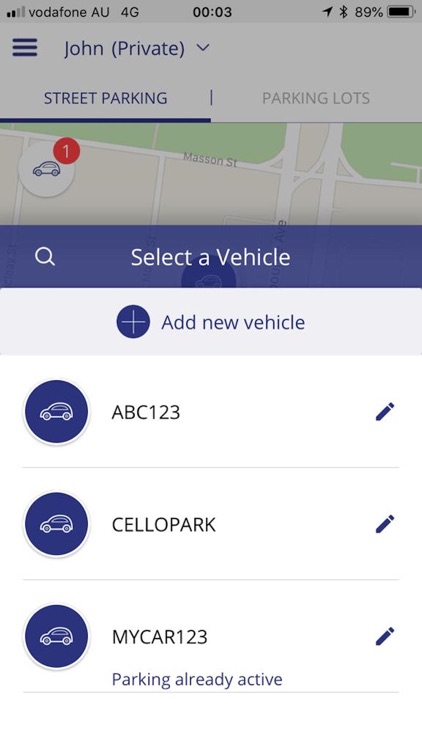At 3 minutes past midnight, the screen displays an app interface with an 89% battery level. The app's header reads "John Private Free Parking" with a map shown underneath. A prominent search bar allows users to select a vehicle, and an "Add New Vehicle" button is available below it. The app's theme is predominantly dark navy blue. 

Three vehicles are listed:
1. "ABC123"
2. "CelloPark" (spelled C-E-L-L-O-P-A-R-K)
3. "My Car 123"

Beneath the "My Car 123" entry, a message notes that parking is "already active." On the right side of each vehicle entry, there is an edit icon allowing modifications to the respective vehicle details.